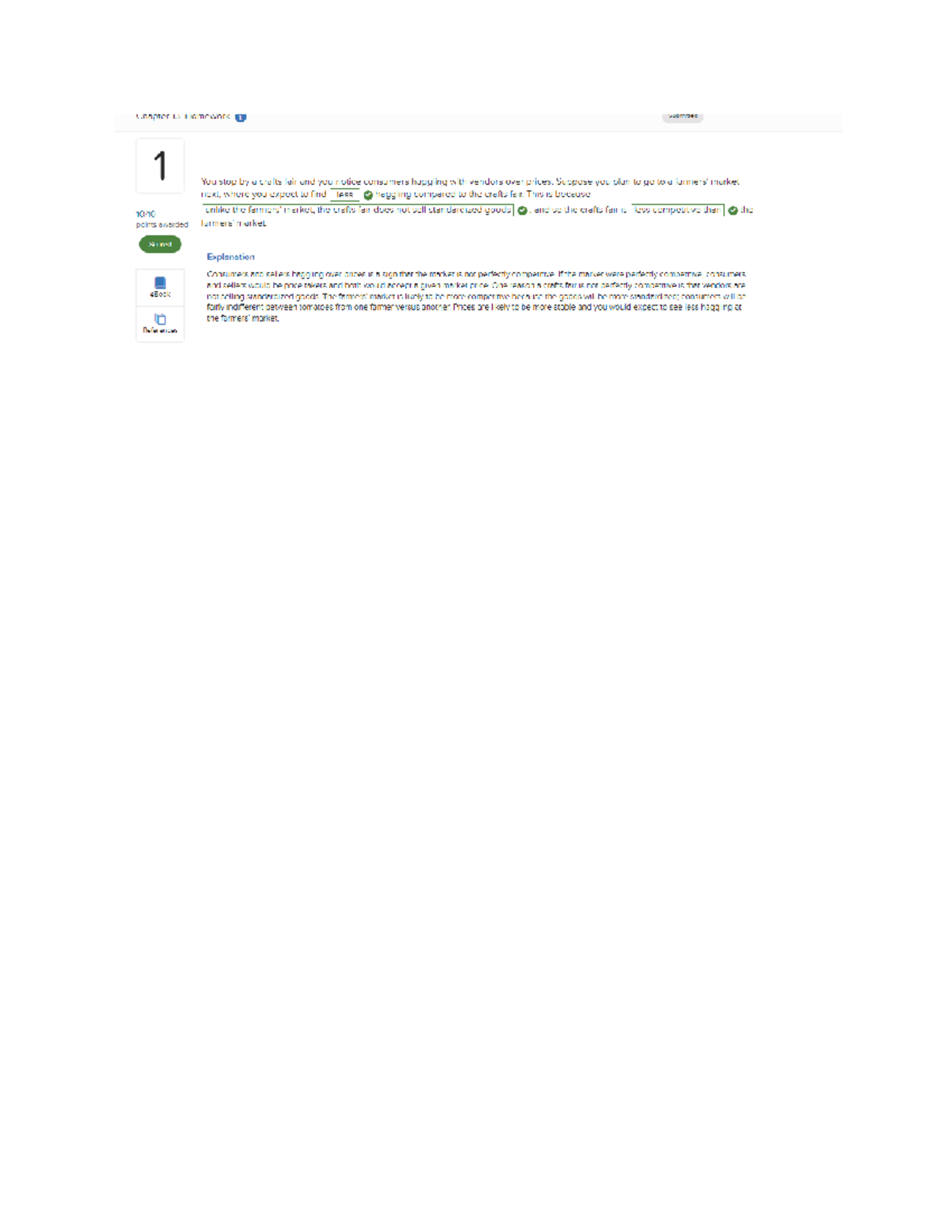This is a small rectangular image with its longer side oriented horizontally. A border runs along the top of the image but contains text that is illegible. Below this border, the image is divided into two sections: a column on the left and a wider section on the right. In the left column, there is a prominently displayed number "1" followed by a green oblong circle featuring white text that is unfortunately unreadable. Adjacent to the number and the green circle are small icons, one resembling a computer and another mimicking a file. To the right of this column, in the larger section, there is a cluster of words. The only discernible piece of text among these words is a title, although the specifics of the title are not clear.